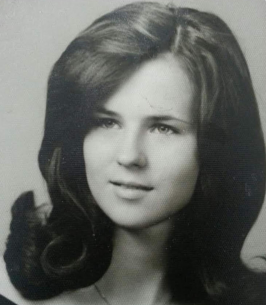This is a small, vertical rectangular black-and-white photograph that appears to be several years old, resembling a high school yearbook picture from the 1960s. The image features a young woman in her late teens or early twenties with very long, dark hair that is parted slightly to her left side, cascading down and curling at the ends as it rests on her shoulders. Her hair partially covers one side of her face, slightly obstructing her vision from one eye. She gazes thoughtfully just off to the side rather than directly at the camera, with light-colored eyes and a slight smile, her lips slightly parted. She is wearing what appears to be a drape that reveals her neck and the tops of her shoulders, along with a delicate chain necklace. The backdrop is a solid medium gray, setting a neutral tone and focusing attention on her features.